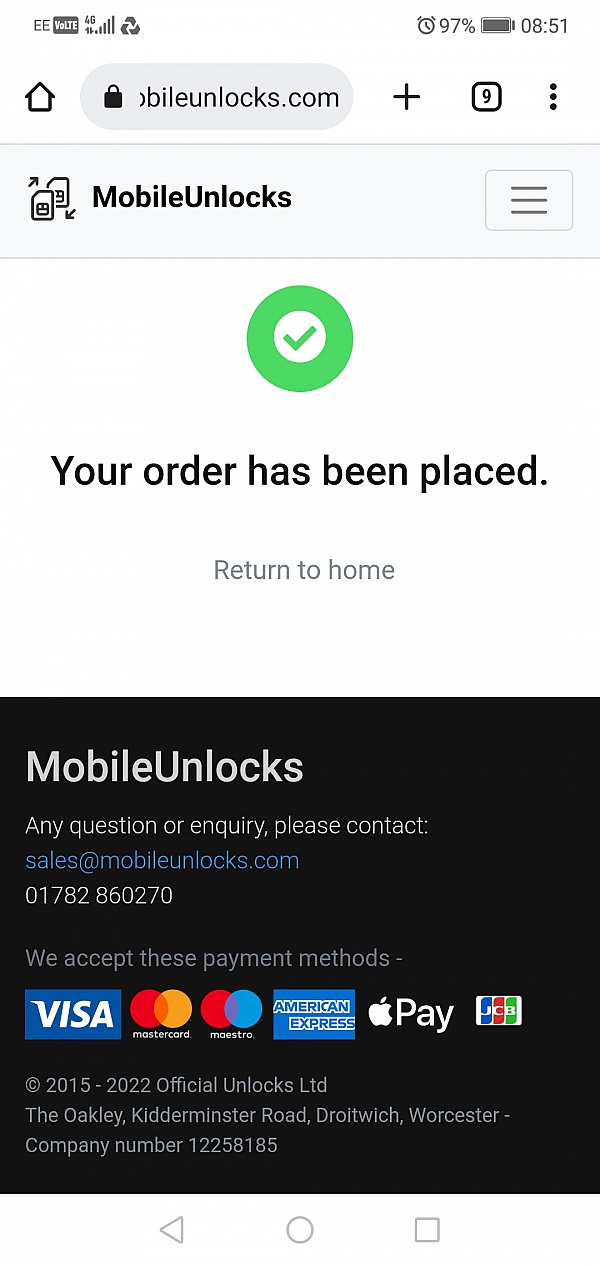This image depicts a screenshot of an Android phone's screen. In the top-left corner, the status bar displays the carrier name "EE" followed by "VoLTE" and a "4G" network symbol, indicating strong connectivity. Adjacent to these, a five-bar signal icon confirms good cellular reception. Additionally, there is a three-arrow recycling symbol, resembling a clover, visible on the screen.

On the upper right-hand side, an alarm clock icon is visible next to a battery percentage indicator showing 95%, coupled with the time, 8:51. The main content of the screenshot presents a website, mobileunlocks.com. A header banner at the top of the webpage displays the site's name, "Mobile Unlocks," alongside three horizontal lines signifying a dropdown menu.

In the center of the page, there is a prominent green checkmark enclosed in a white and then green circle, symbolizing a completed action. Beneath this icon, the message "Your order has been placed" is clearly visible, followed by a "Return to Home" button.

At the bottom of the webpage, the text reiterates "Mobile Unlocks." It also provides contact information for inquiries or support, listing an email address, sales@mobileunlocks.com, and a phone number, 017-828-60270.